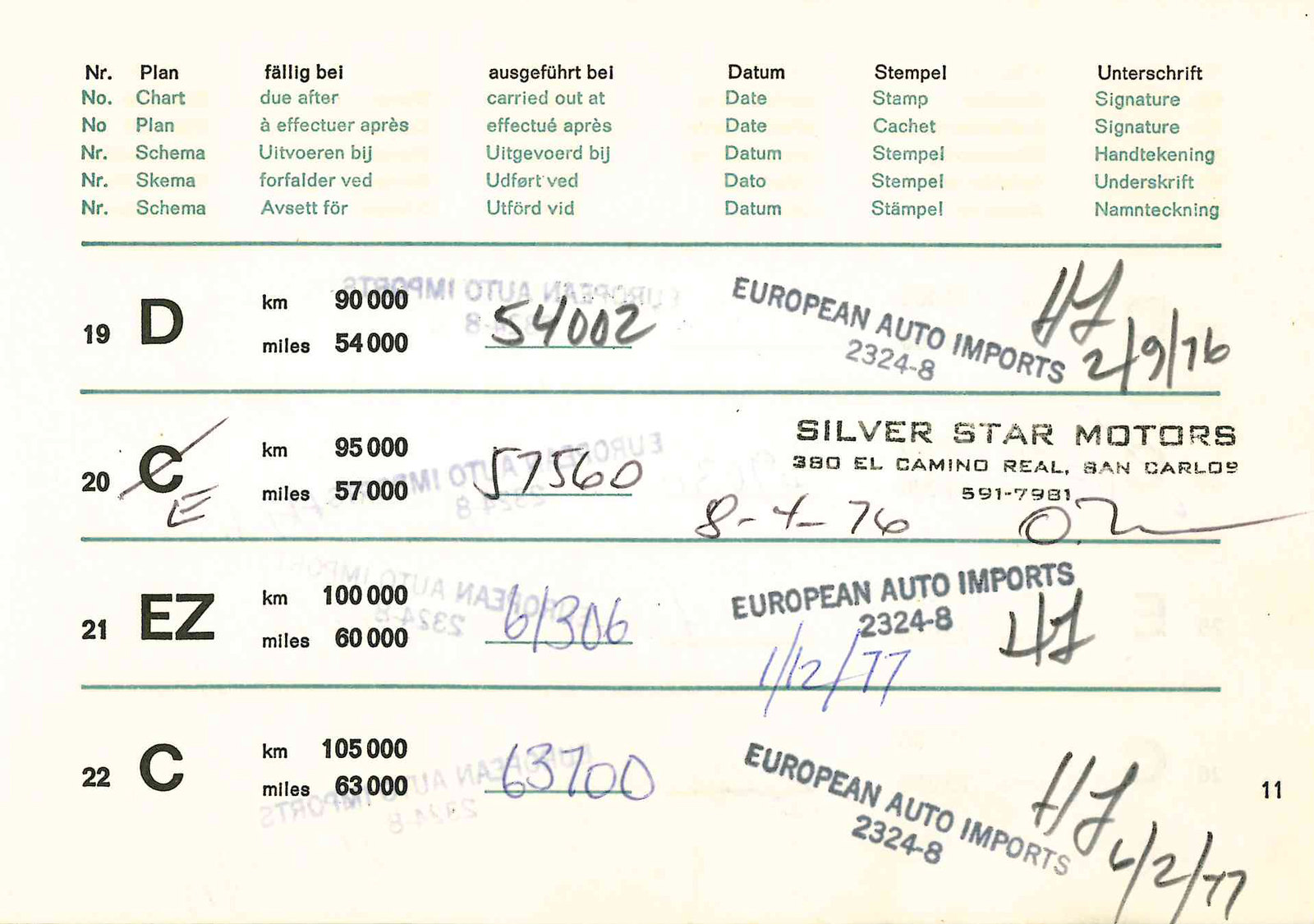The image depicts a detailed automotive maintenance log, resembling a slightly larger than postcard-sized document, possibly a color photo or a photo of a photocopy. The top section appears to organize the layout with headings such as "Number Plan," "Chart," "Schema," "Date," "Stamp," and "Signature." Below, the document tracks maintenance activities for a vehicle, documented in kilometers and miles, with corresponding dates and signatures. 

- **Row 1 (19-D)**: Indicates a service at 90,000 kilometers (54,000 miles), recorded as 54,002 miles, stamped by European Auto Imports on 29/76 with the service provider's signature.
  
- **Row 2 (20-E)**: Lists 95,000 kilometers (57,000 miles) with an actual mileage of 57,560, serviced by Silver Star Motors on El Camino Real, San Carlos, dated 8/4/76 and signed.

- **Row 3 (EZ)**: Documents a service at 100,000 kilometers (60,000 miles), showing a recorded mileage of 61,306, stamped by European Auto Imports on 11/2/77 with the signature.

- **Row 4 (22-C)**: Notes a service at 105,000 kilometers (63,000 miles), recorded as 63,700 miles, stamped by European Auto Imports on 6/2/77, and signed.

The document uniquely integrates handwritten annotations, stamps, and signatures to validate each service entry, emphasizing its meticulous record-keeping of the vehicle's maintenance history.